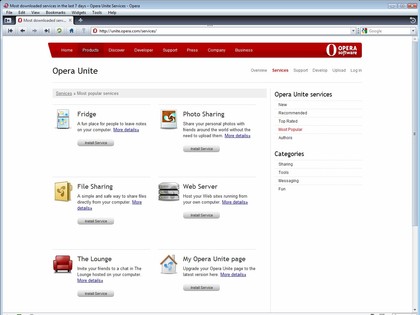The image displays a screenshot of a web browser interface. At the top of the screen is a somewhat blurry address bar. Below the address bar, there is a prominent red header that contains clickable menu items, including the word "Opera" accompanied by its iconic "O" logo. Just beneath this header, the text reads "Opera Unite."

On the right side of the screen, several menu options are visible, including "Overview," "Services," and "Support." Below these options, several icons and their corresponding labels are displayed vertically. These include:

- A refrigerator icon labeled "Fridge"
- An icon for file sharing
- A red sofa icon labeled "The Lounge"
- An icon for photo sharing
- A house with a chimney icon labeled "Web Server"

The bottom section of the interface shows the text "My Opera Unite Page" with a heading next to it that reads "Opera Unite Services." Below these sections, there is an additional label that reads "Categories."